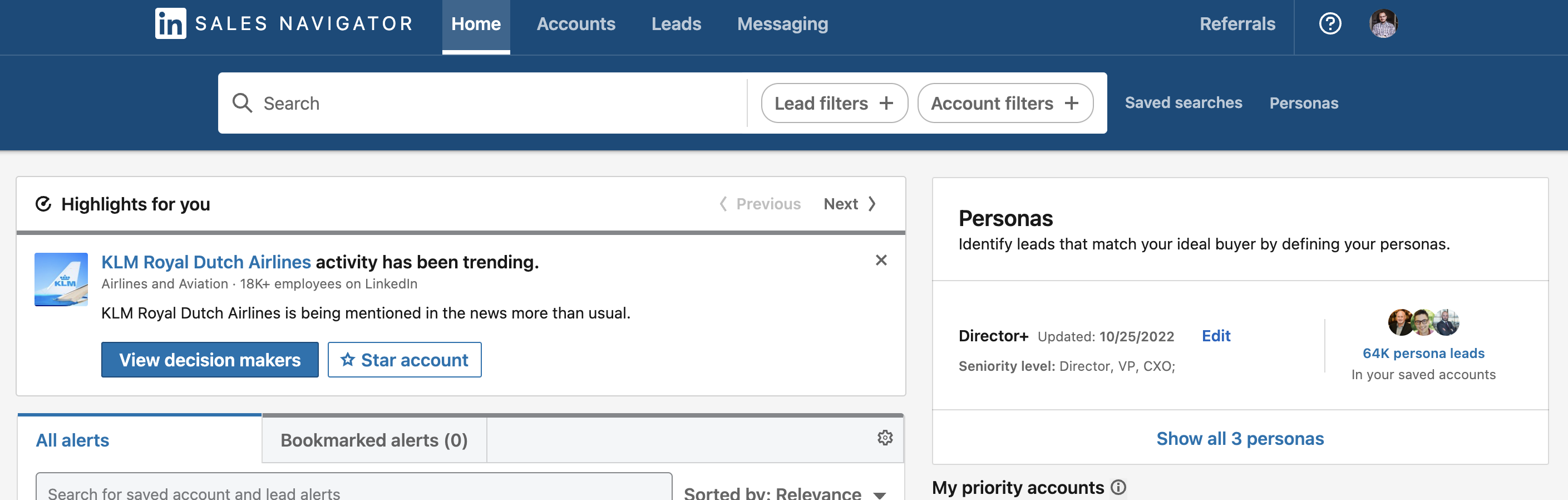The image depicts a webpage of a tool called "IN Sales Navigator." In the upper-left corner, the title "IN Sales Navigator" is prominently displayed within a blue bar. Below this, there is a substantial white search bar spanning horizontally, and to its right, options labeled "Lead Filters" and "Account Filters."

Beneath the search bar, the layout transitions to a gray and white rectangular section. In the upper left of this section, the text "Highlights for you" is written in black. Adjacent to this, there is an image of the tail of a plane, marked with "KLM, Royal Dutch Airlines." Text near the image states that KLM has seen a spike in media activity, noting that the airline is being mentioned in the news more frequently than usual. A blue box labeled "View Decision Makers" is clickable and has been selected.

Further down, a section titled "All Alerts and Bookmark Alerts" shows a count of zero alerts. To the right of this, another rectangular area in white with black text includes information on "Personas." This section explains the feature of identifying leads that match the user's ideal buyer personas. There are three small, circular images of people, representing the personas, with a text indicating "64K persona leads in your saved accounts." At the very bottom, a blue clickable text states "Show all three personas."